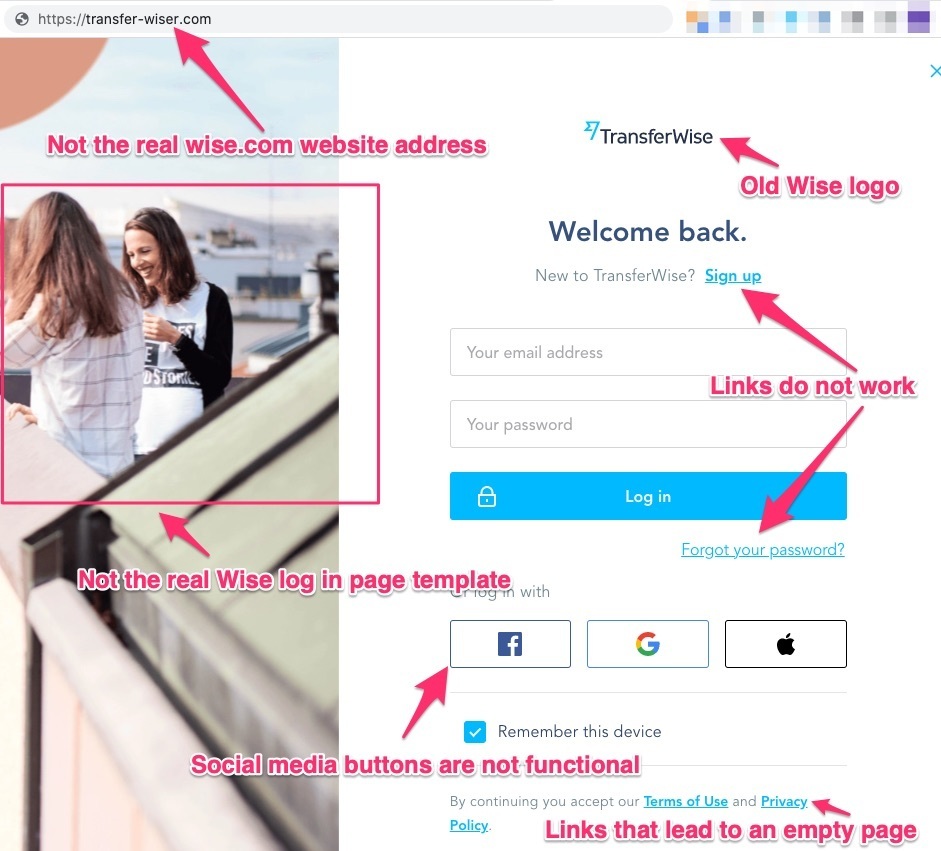The image depicts what appears to be a fraudulent website or app, designed to mimic the legitimate TransferWise (now Wise) service. Key elements include:

1. **URL Indication:** In the upper left-hand corner, the URL reads "https://transfer-wiser.com" with an extra hyphen between "transfer" and "wiser," indicating it is not the official Wise website.
2. **Visual Alert:** A red arrow points to the suspicious URL to draw attention.
3. **Imagery:** Below the URL, there is a photo of two women, one of whom is smiling.
4. **Login Page Facade:** The page is designed to resemble a login page, but it is noted that it is not the real Wise login template.
5. **Social Media Icons:** Icons for Facebook, Google, and Apple are present, suggesting the possibility of signing in via these platforms, though the buttons are non-functional.
6. **Central Elements:** At the center of the page, the old TransferWise logo and the text "Welcome back" are displayed. Links for "I'm new to TransferWise" and "Sign up" are also present, yet a red arrow indicates these links are broken.
7. **Footer Disclaimer:** Towards the bottom of the page, there is text stating "By continuing you accept our Terms of Use and Privacy Policy," with another red arrow pointing out these links as well, which lead to empty pages.

Overall, the image serves as a warning against a phishing site attempting to deceive users into believing it is the authentic TransferWise (Wise) platform.